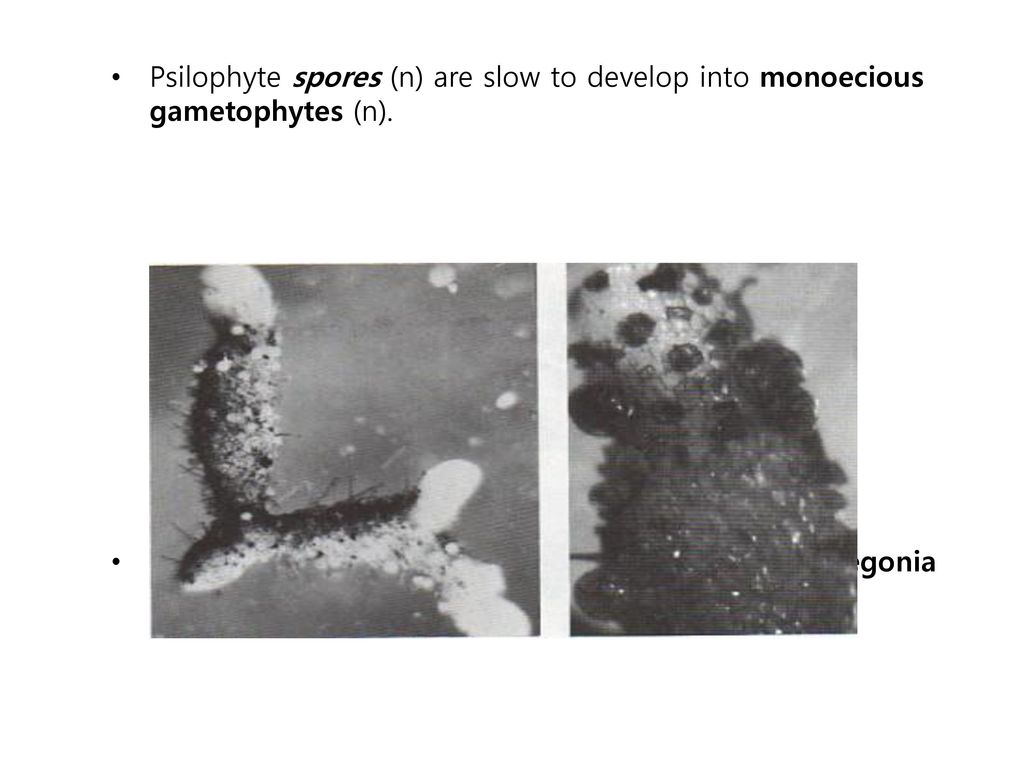The image appears to be an excerpt from a scientific textbook, featuring two black and white microscopic photographs accompanied by descriptive text. The caption, formatted in a bullet point, reads: "Silophyte spores (noun) are slow to develop into monoecious gametophytes (noun)." Key terms such as spores, monoecious, and gametophytes are emphasized in bold. The text introduces two photographs, which are positioned below the description. The photograph on the left showcases a Y-shaped silophyte spore with hair-like structures protruding from it, and dark granular pigments suspended in a lighter matrix. The image on the right depicts a cylindrical spore covered in small black spherical pores. Partially visible text behind this image appears to end with "gonia," possibly indicating a term cut off in the printing.